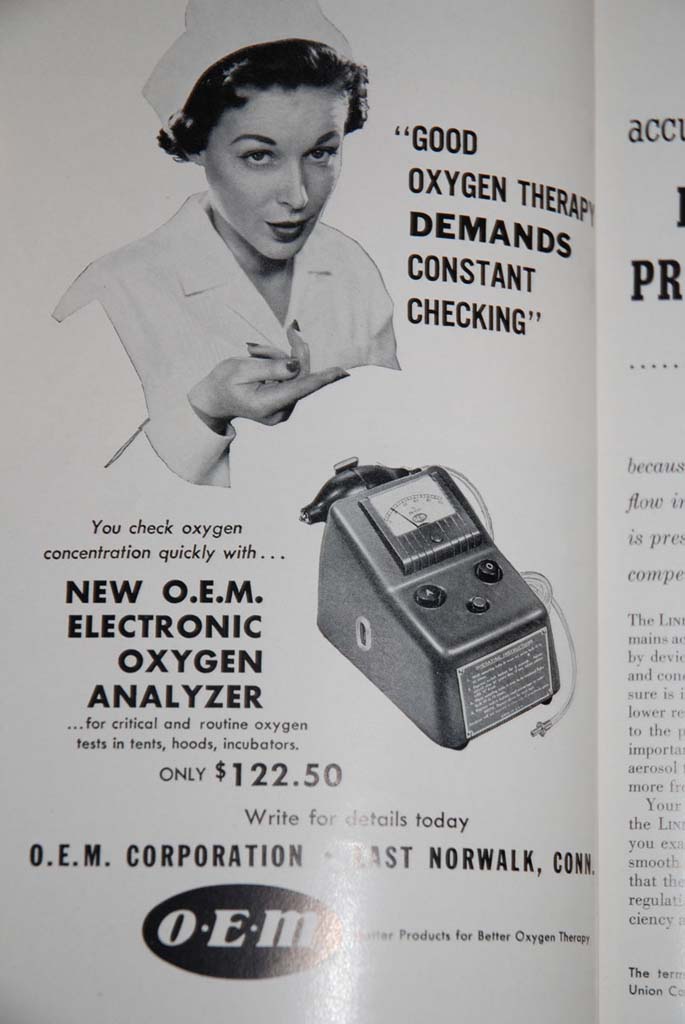The black and white photograph appears to be an advertisement from the 1950s, likely featured in an old magazine. The main focus of the ad is on the left page, with a faint glimpse of the adjacent page on the right. At the top of the page, there is an image of a nurse with short curly hair, dressed in a white uniform and nurse's cap, pointing to a text that reads, “Good oxygen therapy demands constant checking.” Below this, there is a detailed image of an electronic oxygen analyzer, which features three buttons, a small screen with an arrow resembling a clock hand, and a meter. The accompanying text to the left of the device states, “You check oxygen concentration quickly with new OEM electronic oxygen analyzer for critical and routine oxygen tests in tents, hoods, incubators. Only $122.50. Write for details today, OEM Corporation, East Norwalk Con.” At the bottom of the image, the OEM logo is displayed in a white text on a black oval, captioned with, “products for better oxygen therapy.” A slight glare from light reduces the readability of some finer details at the bottom.